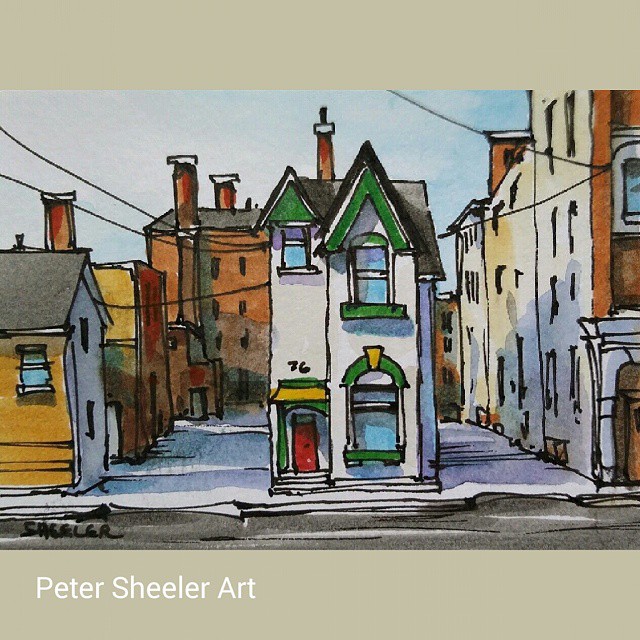The artwork, titled "Peter Sheela Art," is a mixed media piece by Peter Sheeler, combining ink outline drawings and watercolour fills. The image primarily focuses on a central two-story residential building with the number 76, featuring a dominant white facade accented by green-bordered windows and a red door. The door is topped with a bright yellow canopy. The steeply angled gray roof is complemented by a brown chimney with a black pipe. Flanking the building are two large alleyways, and the skies above feature a vivid blue background with a single large white cloud. The illustration, outlined with thick black ink and colored in watercolour, portrays an urban setting with multiple residential buildings, including those in the background which are depicted in orange and browns. Black lines in the sky suggest electricity lines, adding to the urban feel. The entire composition has a slightly cartoony style, with a mix of detailed and suggestive elements to convey the vibrant urban landscape.